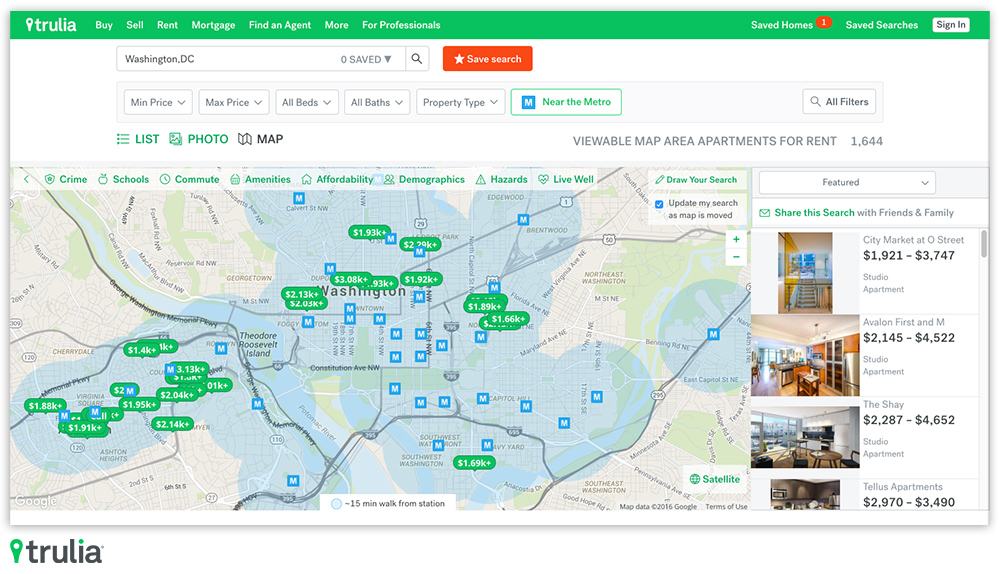Screenshot Description:
The image showcases a desktop screenshot of the Trulia website, identifiable by its green map pin logo. The website's navigation bar, from left to right, includes options for Buy, Sell, Rent, Mortgage, Find an Agent, More, and For Professionals. Additionally, there are links for Saved Homes (highlighted by a notification bubble indicating one saved home), Saved Searches, and Sign In, all encased in a green bar featuring white text.

Central to the page is a search bar pre-filled with "Washington DC, zero saved," alongside a prominent red box with white text labeled "Save Search." Directly below are various filtering options allowing users to set preferences for Minimum Price, Maximum Price, number of Beds, number of Baths, Property Type, and proximity to the Metro. An "All Filters" option offers further customization.

The next section presents viewing options such as List, Photo, Map to explore the area. Underneath this are details indicating there are 1,644 apartments available for rent in the Washington DC area, displayed on a detailed map punctuated by different price points.

Users can filter their search results based on categories like Crime, Schools, Commute, Amenities, Affordability, Demographics, Hazards, and Live Well. Trulia provides interactive features, such as the ability to draw a custom search area and an "Update my search as map is moved" option. The map is adjustable between standard and satellite views, with zoom capabilities.

To the right of the main content, the site highlights featured listings and provides the option to "Save this search with friends and family." Featured listings include:
- City Market at O Street: Studio apartments ranging from $1,921 to $3,747 per month.
- Avalon First and M: Apartments priced between $2,145 and $4,522 per month.
- The Shea: Studio apartments costing from $2,287 to $4,652 per month.
- TELUS apartments: Listings between $2,970 and $3,490 per month.

The detailed screenshot serves as a guide for navigating Trulia’s interface and exploring real estate options in Washington DC.